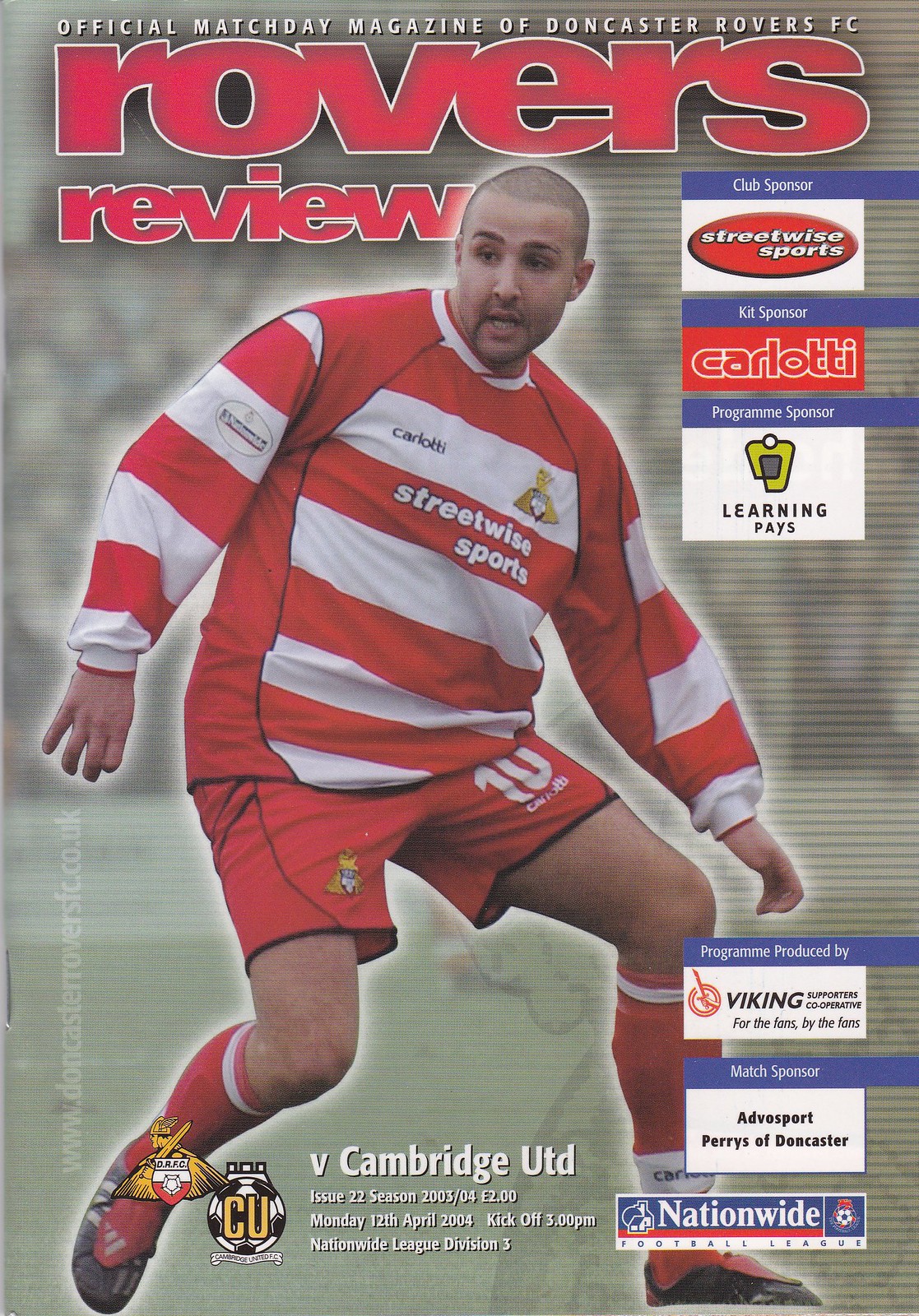This is the front cover of a soccer program, likely for a British football club. The title "Rovers Review" dominates the top, "Rovers" in red lowercase letters spans the width from left to right, with "Review" slightly smaller and left-justified beneath it. The background depicts a blurred crowd with indistinct, white roundish figures, enhancing the focus on the foreground subject.

The main image features a slightly heavyset Caucasian gentleman with a near-shaved buzz cut and dark hair, looking slightly to his right as he stands on a pitch. He sports a long-sleeved red and white horizontally striped jersey with "Streetwise Sports" in white lowercase font across one of the stripes. His red shorts are marked with the number "10" in white on the left thigh, and he wears red socks with a single white stripe near the top, paired with black boots. Positioned as if preparing to engage with the ball, he has both legs bent; his right foot is partially lifted, with toe touching the ground and heel raised.

Down the right side of the cover, there is a column of small advertisements, listing sponsors such as Club Sponsor, Kit Sponsor, Program Sponsor, and specific names like Streetwise Sports, Carlotti, Learning Pays, Viking, Advo Sport, Perry's of Doncaster, and Nationwide at the bottom. The lower center of the cover states "V. Cambridge UTD," with "Cambridge UTD" to the left, adjacent to a symbol with gold letters "CU." The issue details at the bottom mention the price of two pounds, the date April 2004.